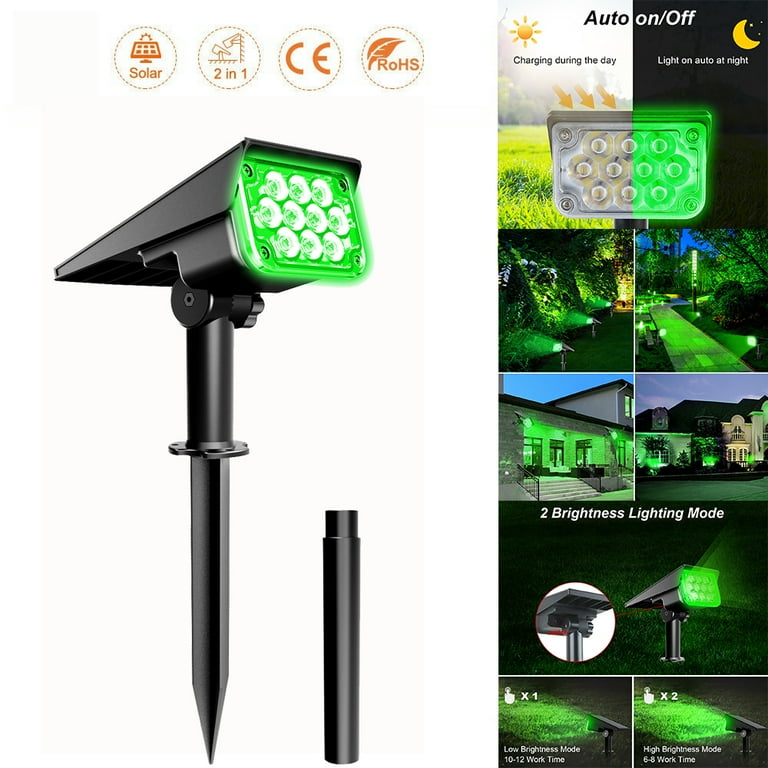The image is an advertisement for a versatile solar-powered lighting system designed for outdoor landscapes. The main focus is on a solar light with a solar cell on top that charges during the day and automatically illuminates at night. This innovative light, which features a vibrant green hue due to a filter, can be assembled from several pieces and conveniently staked into the ground. The system includes ten bulbs and offers two brightness modes, making it suitable for both residential and business use. Accompanying the text "charging during the day, light on auto at night," the advertisement features a series of small images displaying various applications of the lights, such as highlighting pathways, steps, lawns, and building facades. These images demonstrate how the solar lights, unobtrusive during the day, provide depth and illumination to outdoor spaces once the sun sets.